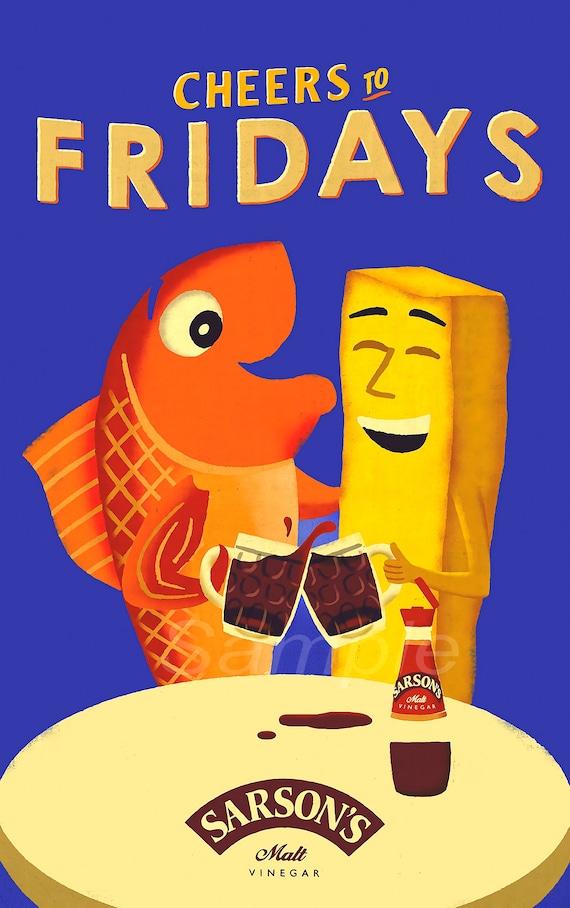The image is an advertisement for Sarson's Malt Vinegar featuring a vibrant, playful design set against a blue background. At the top, bold yellow lettering in uppercase reads "Cheers to Fridays," with the word "TO" underlined in orange for emphasis. Below the text, two cartoon characters—a human-like orange fish and a yellow, stick-like figure that resembles a french fry—are toasting each other with mugs filled with a brown liquid, likely malt vinegar. Both characters have cheerful expressions, and the fish is standing upright, holding its glass with a fin, while the french fry character uses a human-like arm. These anthropomorphic characters are positioned beside a yellow table, which has a bottle of Sarson's Malt Vinegar on it. The bottle is half-empty, clear with a red label and white lettering spelling out "Sarson's." Some of the vinegar appears to have spilled on the table. The Sarson's logo is displayed on a curved brown banner with light yellow writing, reinforcing the branding. This lively scene captures a celebratory moment, illustrating the fun and zest of enjoying Sarson’s Malt Vinegar on a Friday.